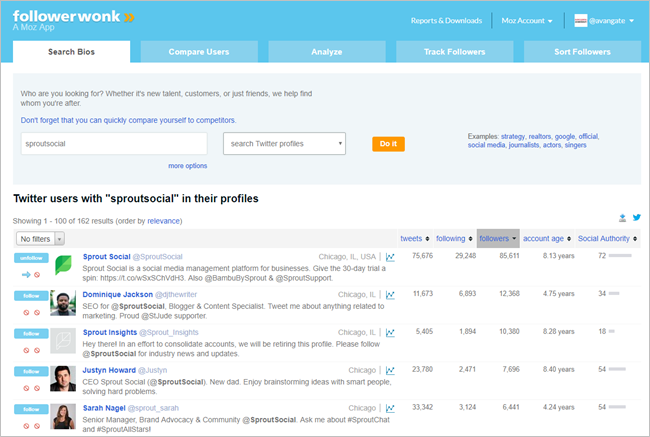At the top of the page, a sky-blue colored border features the heading "Follower Walk, a Moz app." To the right, there are options labeled "Reports and Downloads," "Moz Account," and "Avangate" next to a profile icon. Below the border, several selectable tabs are available: "Search BIOS," "Compare Users," "Analyze," "Track Followers," and "Sort Followers," with "Search BIOS" currently selected.

The interface prompts with "Who are you looking for? Whether it's new talent, customers, or just friends, we're here to help you find whom you're after. Don't forget that you can quickly compare yourself to competitors." Beneath this, a text box labeled "Search Twitter Profiles" contains the term "Sprout Social," accompanied by an orange button labeled "Do It."

Below the search box, the results section titled "Twitter Users with Sprout Social in their profiles" displays 1 through 100 of a total of 162 results. The top results include "Sprout Social," "Dominique Jackson," "Sprout Insights," "Justin Howard," and "Sira Nagel." Each user profile is listed with categories such as "Tweets," "Followings," "Followers," "Account Age," and "Social Authority," with corresponding data presented for each individual.